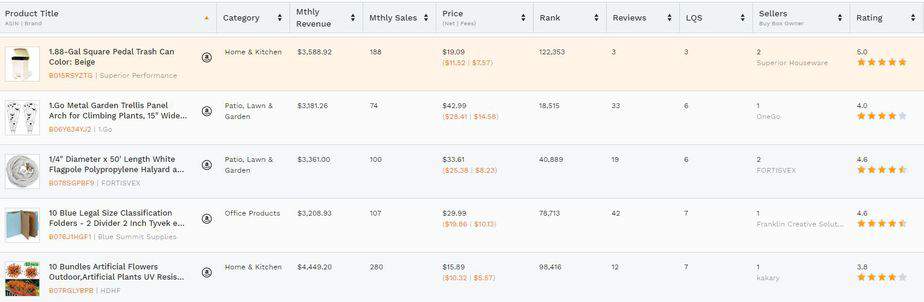Here's a detailed and cleaned-up caption for the image described:

---

Screenshot of a data table listing various product metrics. The table headers include: Product Title, Category, Monthly Revenue, Monthly Sales, Price, Rank, Reviews, LQS (Listing Quality Score), Sellers, and Rating. Each header is accompanied by up and down arrows, indicating sortable columns.

The first row of the table features product information within a highlighted red rectangle, while subsequent rows display alternating light gray and gray backgrounds.

1. **Product Title:** Oval/Square Petal Trash Can  
   **Category:** House and Kitchen  
   **Monthly Revenue:** Blurred (amount not visible)  
   **Monthly Sales:** 156 or 155 (uncertain)  
   **Price:** Blurred (amount not visible)  
   **Rank:** Blurred  
   **Reviews:** 3  
   **LQS:** 3  
   **Sellers:** 2  
   **Rating:** 5 stars  

The next item in the list is titled "Gold Medal Garden Trellis Panel - Arch for Climbing Plants."

---

This caption provides a structured and comprehensive overview of the image content, making it easy to understand at a glance.